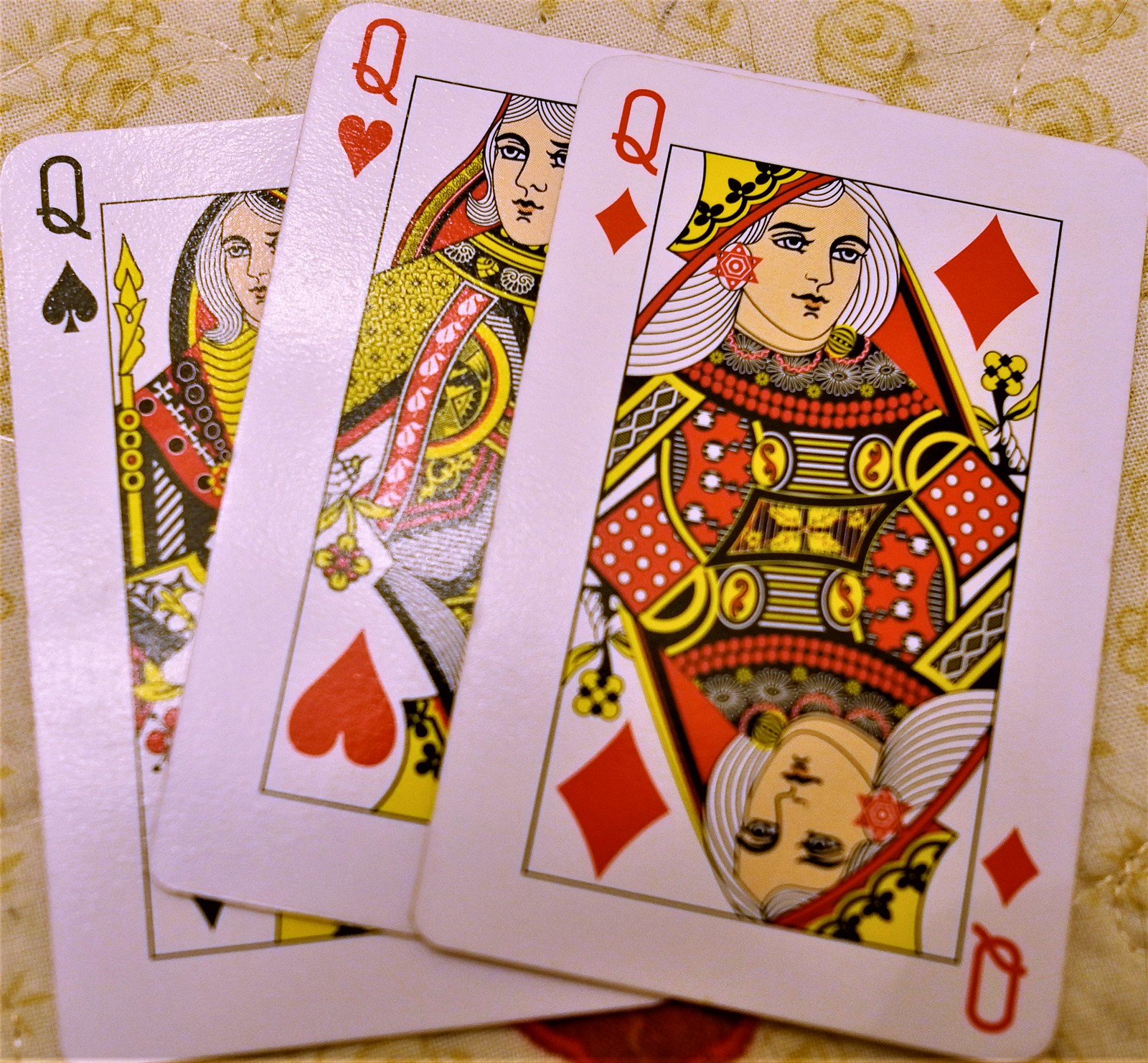In the image, there are three standard playing cards arranged in a spread. The bottom card is the Queen of Spades, the middle card is the Queen of Hearts, and the top card is the Queen of Diamonds. These cards, typically seen in casinos, have a white background and display images of queens. Each card features a queen adorned in a patterned dress and crown, with a mirror image of the queen below the original. The cards are laid out on a beige cover that resembles upholstery, adorned with a flower pattern outlined in yellow. The cover shows visible stitching, adding to the texture and detail of the background.